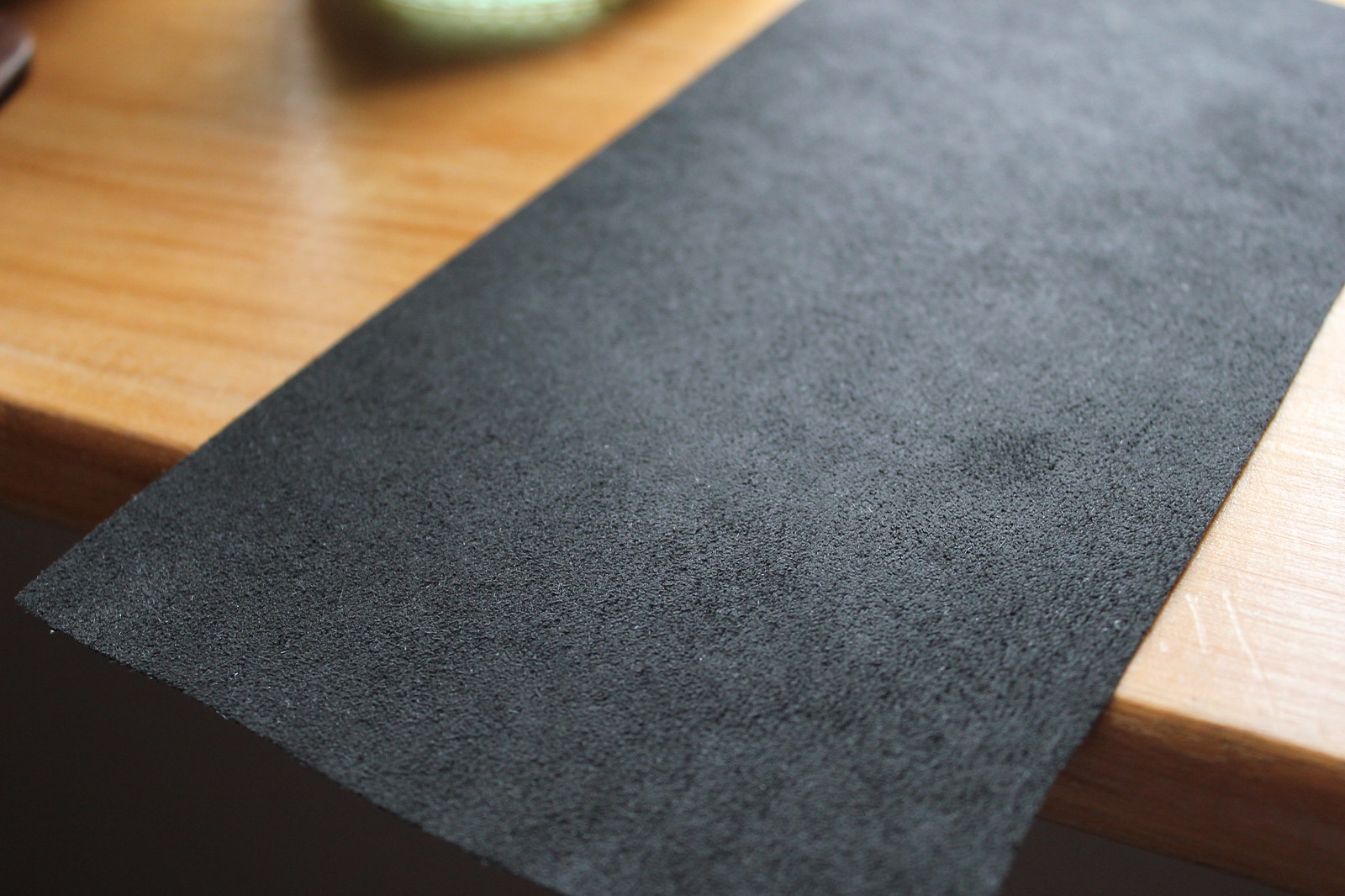The indoor photograph captures a scene where a black strip, possibly made of rubber or vinyl, is laid out on the surface of a medium-toned wooden table. The strip, textured and somewhat stiff, extends diagonally from the lower left to the upper right edge of the frame, with a small portion hanging off the table's edge. The table's wood grain runs diagonally, from the upper left to the lower right. Notably, there are three small scrapes in the wood where the black strip meets the right edge of the table. The background reveals a mysterious green glowing object, which could be either on the table or a reflection from above, although its exact source is indiscernible from this angle. The overall dimensions of the photograph include roughly a four-inch height and a six-inch width, creating a close-cropped view that leaves the full length of the black strip outside the frame, hinting at its considerable length.